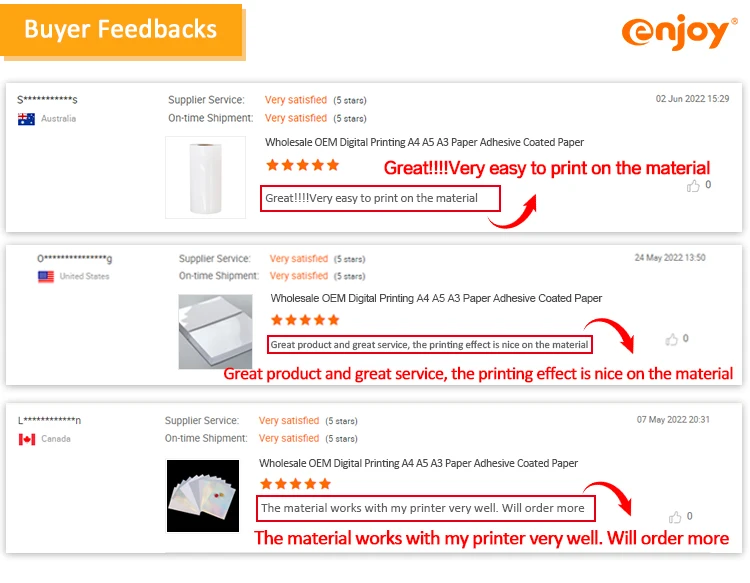This image is a section for buyer feedback on a website called Enjoy. The Enjoy logo is positioned in the upper right corner, featuring a white "E" in negative space, surrounded by an orange swirl. The letters "njoy" are displayed in lowercase to the right of the "E," accompanied by a small registered trademark "®" symbol above the "y."

The image contains three floating panels with drop shadows, each showcasing customer reviews. Overlaid on these panels are red text, arrows, and lines highlighting specific areas of interest.

1. **First Panel (Australia)**
   - **Anonymous Reviewer from Australia**
   - **Supplier Service**: Very Satisfied (5 stars)
   - **Online Shipment**: 5 stars
   - **Product Details**: Wholesale OEM, digital printing, A4, A5, A3, paper adhesive, coated paper 
   - **Image**: Roll of paper standing vertically
   - **Feedback**: "Great, very easy to print on the material!!!!"
   - This feedback is emphasized with a red arrow pointing to a quote in large red text over the top of the panel.

2. **Second Panel (United States)**
   - **Anonymous Reviewer from the United States**
   - **Supplier Service**: Very Satisfied
   - **Online Shipment**: Very Satisfied 
   - **Product Details**: Wholesale OEM, digital printing, A4, A5, A3, paper adhesive, coated paper 
   - **Image**: Black and white image of a book
   - **Feedback**: "Great product and great service. The printing effect is nice on the material."
   - This comment is similarly highlighted with a red arrow and an enlarged red text overlay.

3. **Third Panel (Canada)**
   - **Anonymous Reviewer from Canada**
   - **Supplier Service**: Very Satisfied (5 stars)
   - **Online Shipment**: 5 stars
   - **Product Details**: Wholesale OEM, digital printing, A4, A5, A3, paper adhesive, coated stock 
   - **Image**: Fanned out objects, possibly envelopes
   - **Feedback**: "The material works with my printer very well. Will order more."
   - This quote is also accentuated with a red arrow, a red rectangle, and a large red text overlay.